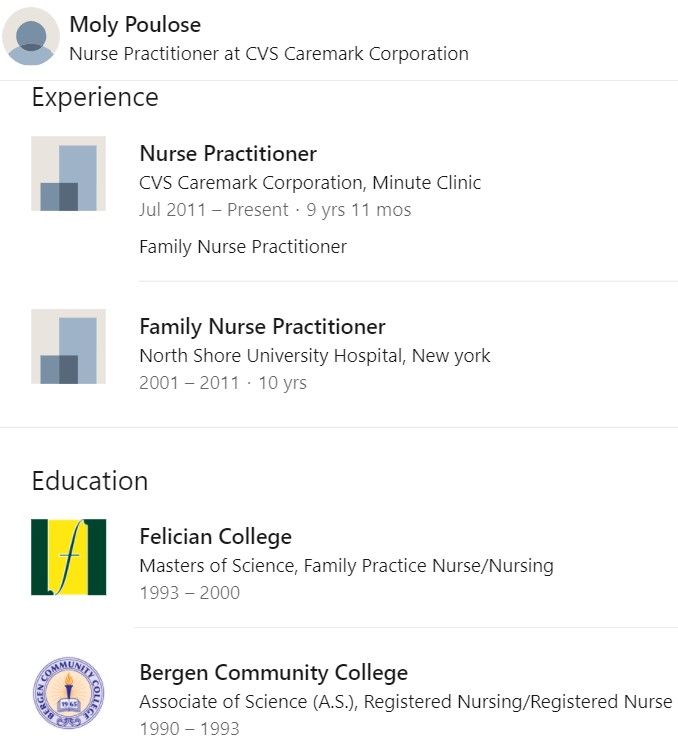The image displays a detailed profile section of a professional website. At the top, the individual's name, Mollie Palouse, is prominently featured. She is identified as a Nurse Practitioner at CVS Karamar Corporation. 

The section is segmented into distinct parts:

1. **Experience:**
   - **Nurse Practitioner, CVS Karamar Corporation, Minute Clinic** (July 2011 - Present): Mollie has served in this role for nine years and eleven months.
   - **Family Nurse Practitioner, North Shore University Hospital, New York** (2001 - 2011).

   A thin gray line divides the Experience section from the Education section.

2. **Education:**
   - **Felician College:** Masters of Science in Family Practice Nurse and Nursing (1993 - 2000). This section is marked with a black and yellow emblem to the left.
   - **Bergen Community College:** Associate of Science (AS) in Registered Nursing and Registered Nurse (1990 - 1993). This section features a purple circle emblem to the left.

The entire profile is set against a clean, white background, allowing each detail to stand out clearly.